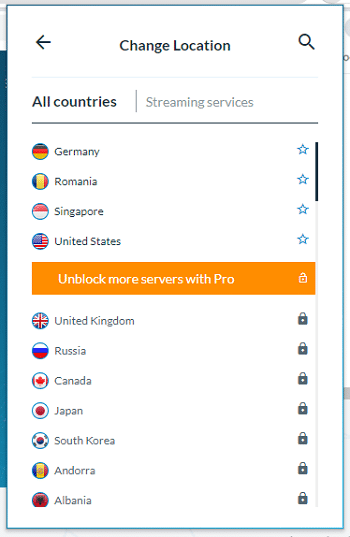A detailed graphical interface screen is displayed. On the left side, there is a back arrow icon. In the center, the text "Change Location" is prominently displayed, followed by a search icon resembling a magnifying glass. Below, the text "All Countries" is visible alongside the label "Streaming Services," which is separated by horizontal lines.

A variety of national flags are presented with associated icons:
- The Germany flag, alongside a hollowed-out star.
- The Romania flag, next to another hollowed-out star.
- The Singapore flag, followed by a hollowed-out star.
- The United States flag, with yet another hollowed-out star.
An orange rectangular button reads "Unblocked Mortars and Probes."

Continuing, the screen shows:
- The United Kingdom flag, accompanied by a gray lock icon.
- The Russia flag (white, blue, red), with a lock icon.
- The Canada flag, next to a lock icon.
- The South Korea flag (red, blue), followed by various marks.
- The Andorra flag (blue, yellow, red), paired with a gray lock icon.
- The Albania flag with its black center and red edges, plus a gray lock icon.

The background features a composition of multiple overlapping window panels against a white backdrop. The foremost window includes a blue segment on the left edge, and faint, partially obscured text is visible. The bottom right corner of this foreground window remains notably gray. The next vertical section shows "All Countries" at the top, separated by a vertical line, with "Streaming Services" in gray text below.